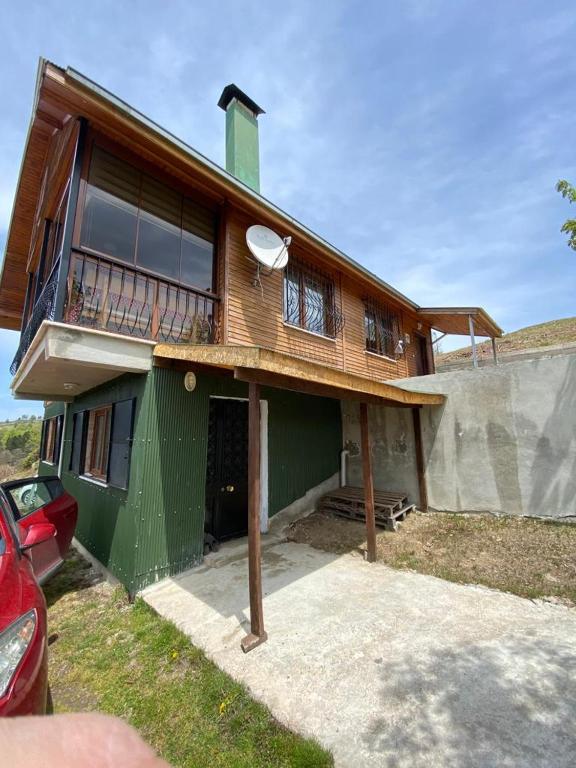This photograph captures a unique, two-story house built on an elevated hill. The bottom level is constructed from green corrugated metal, resembling a shipping container, and features a black front door with a wooden awning overhead. The upper story is composed of natural wood with extensive glass windows, allowing ample sunlight to enter and offering a view outside. The pitched roof is also wooden with green tiles, crowned by a prominent green square chimney. Attached to the upper floor’s wall is a small satellite dish. A red, two-seater car is parked beside the house, partially visible with one door open. The backyard is enclosed by a cloth-like fence and the surrounding area is predominantly flat with dry grass and minimal vegetation, featuring just a single tree and some small bushes. The sky is clear and blue, suggesting a sunny day.